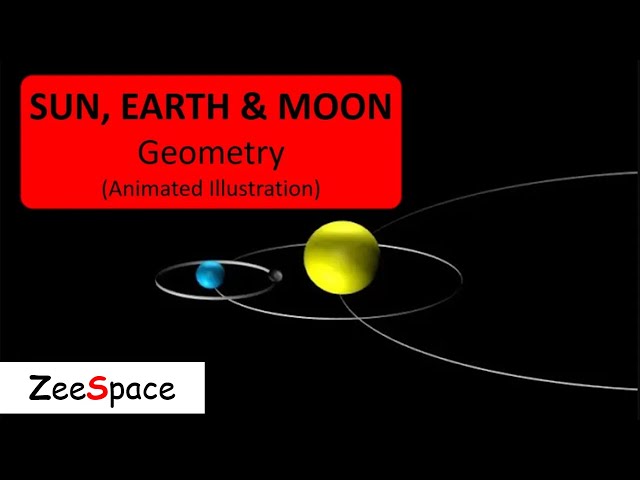The image is a basic 3D representation of part of the solar system. It features a solid black background with two main objects: a very small teal ball, representing the Moon, located on the center-left, and a significantly larger yellow ball, representing the Earth, positioned directly to its right. The teal ball is about 5% the size of the image dimensions, while the yellow ball is roughly eight times larger. Both spheres are encircled by thin, silver rings symbolizing their orbits. A larger half-circle intersects the yellow ball from the right side of the image.

At the top, there is a bold red rectangular box containing the title "Sun, Earth, and Moon Geometry" with "Animated Illustration" noted in parentheses underneath. In the bottom-left corner, another box or strip, this time in white, displays the text "Z Space" in Comic Sans, with the "S" in red and both the "Z" and "S" capitalized. Overall, the illustration is clearly intended to represent the dynamics of the Earth and Moon in relation to their orbits, albeit in a somewhat rudimentary artistic style.